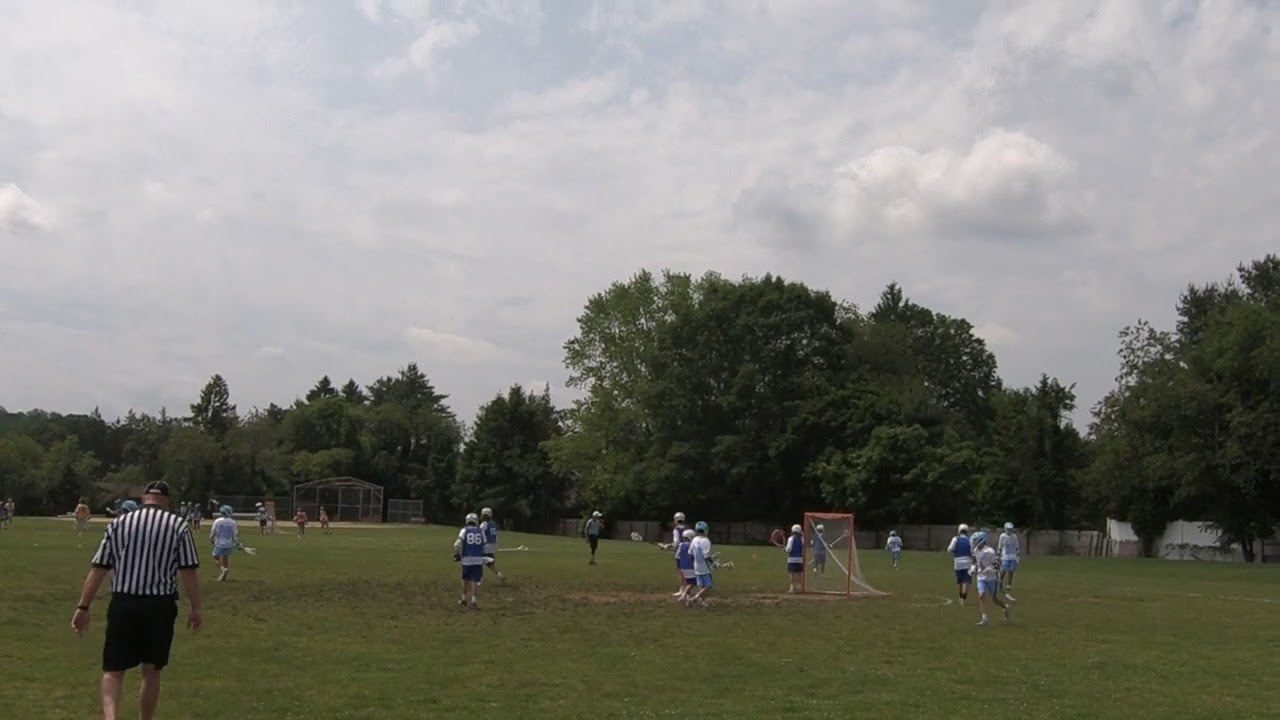The outdoor photograph captures a lively field hockey game on a grassy field. Dominating the lower left corner is a referee, a Caucasian male, clad in the typical black and white striped short-sleeved shirt, black shorts, and a black cap. The scene is set amidst tall, verdant trees that surround the field. The game appears to feature young players, possibly in a peewee league, divided into two teams wearing blue and white jerseys and helmets, indicative of American football, but juxtaposed with hockey sticks and a field hockey net, suggesting a mix-up or unique sporting crossover. Beyond the game, a baseball diamond is partially visible in the backdrop. The sky overhead is coated with thick, white and gray clouds, hinting at an overcast day with sparse patches of light blue sky, adding to the serene yet energetic atmosphere of the game.